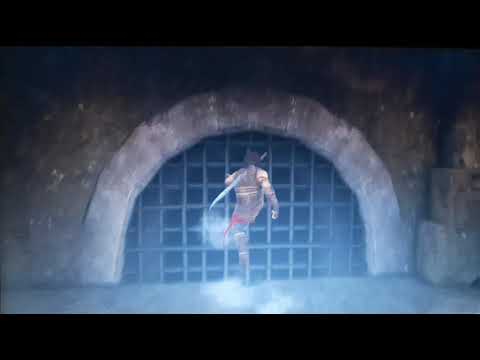In the screenshot of the third-person video game, the player character stands about five or six feet in front of the camera with his back facing it. The scene is framed in a widescreen format, bordered by thin black bars at the top and bottom. The character, dressed as a warrior, wears light, sleeveless armor that features a dark top with a gold belt around the chest, and brownish or possibly blue pants with brown boots. A curved sword is attached to his back, with the handle visible above his right shoulder. He is in the midst of kicking a semi-circular metal sewer grate set into an archway of old, dark grey stone. The grate is surrounded by a semi-circular chunk of concrete. Surrounding the character are various environmental details: to the right, there are wooden pallet-type boxes stacked in a corner. The scene is dimly lit, with the lower portion of the image, particularly around the character's foot on the ground, being significantly brighter, and the lighting gradually darkens towards the top of the image.